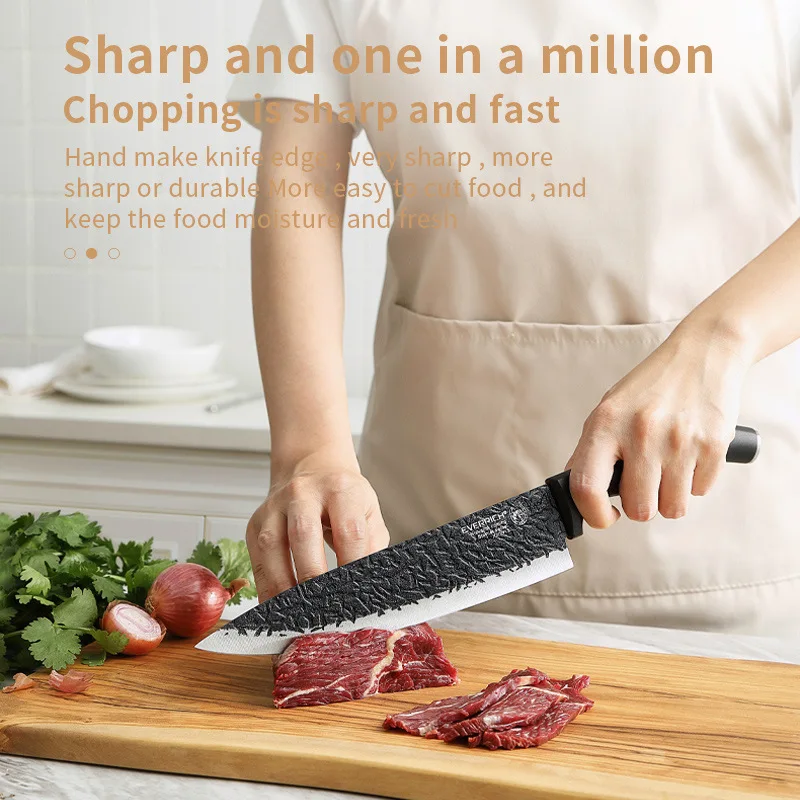The image is an advertisement for a high-quality, handmade chopping knife. It features a close-up of a person chopping fresh beef on a wooden cutting board. The person, who appears to be a woman, is wearing a beige apron over a white t-shirt, although one description mentions a white chef-like smock. Her face is not visible as it is cropped out of the image. She is holding the impressive knife in her left hand while her right hand steadies the beef. Surrounding the beef on the cutting board are a couple of onions and some leafy green vegetables, possibly parsley. Behind the scene is a white kitchen setup with a counter, a white plate holding a white ceramic bowl, and a white wall. Overlaid on the image is marketing text in light brown and orange fonts, proclaiming the knife to be "sharp and one in a million" and promising a "handmade knife edge, very sharp and durable, more easy to cut food and keep the food moist and fresh." The text highlights the knife’s exceptional sharpness and durability, aimed at enhancing cooking efficiency while maintaining food quality. The overall scene underscores the premium nature of the knife, suggesting it is an indispensable tool for any kitchen.